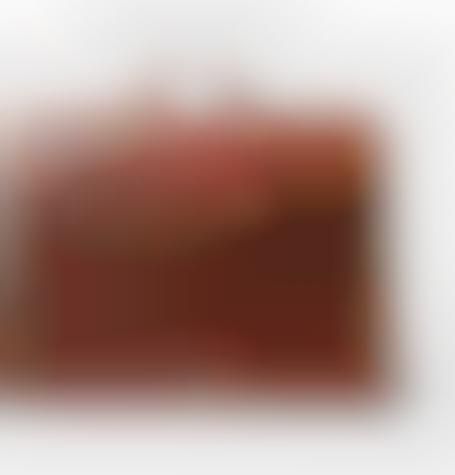The image is predominantly out of focus, making it difficult to discern any specific details. The background of the image is a square that is predominantly white with grayish tones along the upper, lower, and right-hand portions. The central area features a maroon to reddish-brown coloration, which appears hazy and lacks any discernible features. The reddish-brown area seems more intensely colored towards the center and lighter towards the edges, with some lighter red sections above and below the central dark red. Despite the lack of clarity, the central shape vaguely resembles a rectangle or a triangular form, amidst the white-blurred background.